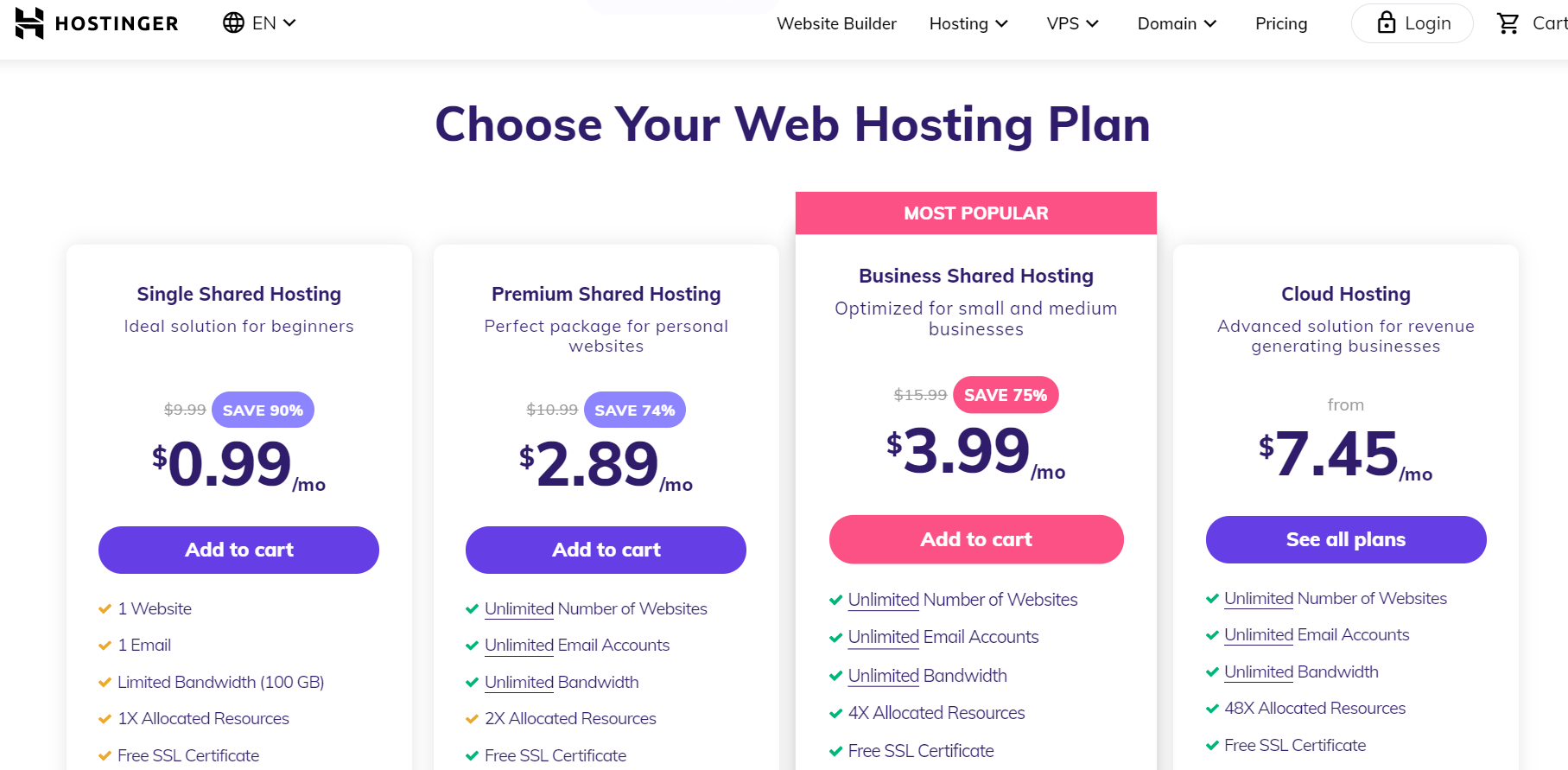This digital image offers a detailed overview of different web hosting plans available from Hostinger, emphasizing their features and pricing. 

1. **Single Shared Hosting**:
   - **Ideal For**: Beginners
   - **Discount**: Save 30%
   - **Price**: $0.99 per month
   - **Features**: 
     - Host one website
     - One email account
     - Limited bandwidth up to 100 GB
     - 1X allocated resources
     - Free SSL certificate
   - **Call to Action**: Add to Cart button present

2. **Premium Shared Hosting**:
   - **Ideal For**: Personal websites
   - **Discount**: Save 74%
   - **Price**: $2.89 per month
   - **Features**: 
     - Unlimited number of websites
     - Unlimited email accounts
     - Unlimited bandwidth
     - 2X allocated resources
     - Free SSL certificate
   - **Call to Action**: Add to Cart button present

3. **Business Shared Hosting** (Most popular option):
   - **Ideal For**: Small and medium businesses
   - **Discount**: Save 75%
   - **Price**: $3.99 per month
   - **Features**: 
     - Unlimited number of websites
     - Unlimited email accounts
     - Unlimited bandwidth
     - 4X allocated resources
     - Free SSL certificate
   - **Call to Action**: Add to Cart button present